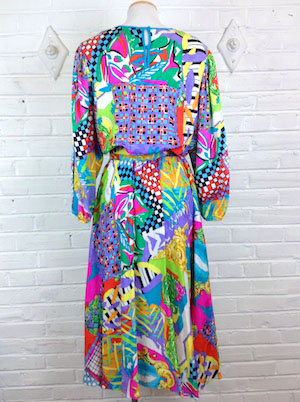This color photograph, presented in a rectangular, portrait orientation, captures the back view of a long-sleeved woman's dress displayed on a headless mannequin with a white fabric body and a brown wooden cap at the neck. The vibrant and colorful dress, characterized by its patchwork of abstract designs, includes checkerboard patterns, cross marks, floral prints, and various lines in shades of lavender, gold, red, pink, purple, green, and blue. The dress is gathered at the waist and has a teardrop opening at the back neckline outlined in blue, with a skirt that flows to around mid-calf or ankle length, depending on the wearer's height. The background of the photograph is a white-painted brick wall adorned with four diamond-shaped patterns, adding to the minimalist aesthetic. The overall scene offers a realistic and detailed portrayal of the dress's intricate designs and vibrant colors.